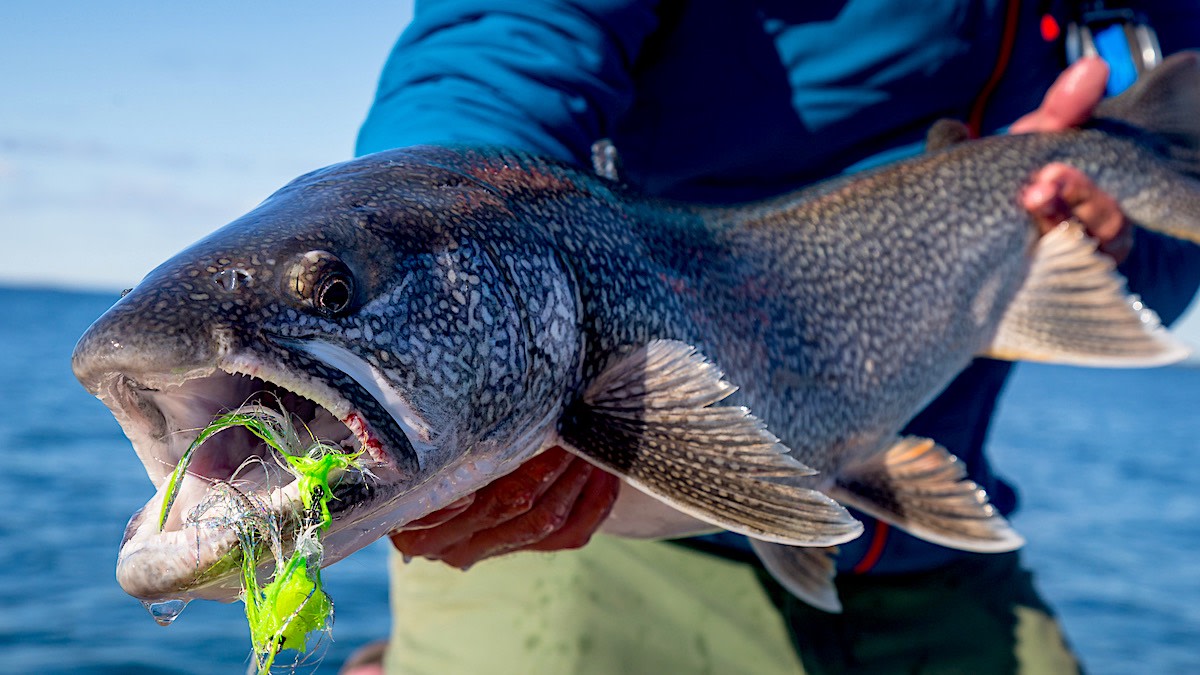In this vibrant color photograph taken on a sunny day, a man stands near a blue lake or ocean, set against a light blue sky. He is wearing a blue jacket or shirt and beige khaki pants. The focal point of the image is the large, speckled lake trout he is holding. The fish, facing the camera with its mouth wide open, reveals a light gray interior and has a bright chartreuse sea plant tumbling out from its mouth. The fish possesses a mottled gray and brown body, smooth in texture, with several visible fins and a bulging eye with a black center. The man supports the fish with his right arm under what would be its neck if it had one, and his left hand positioned just in front of the tail. Some parts of the man's body are cropped out of the photo, leaving the fish as the prominent feature against the serene backdrop of a blue lake and sky.